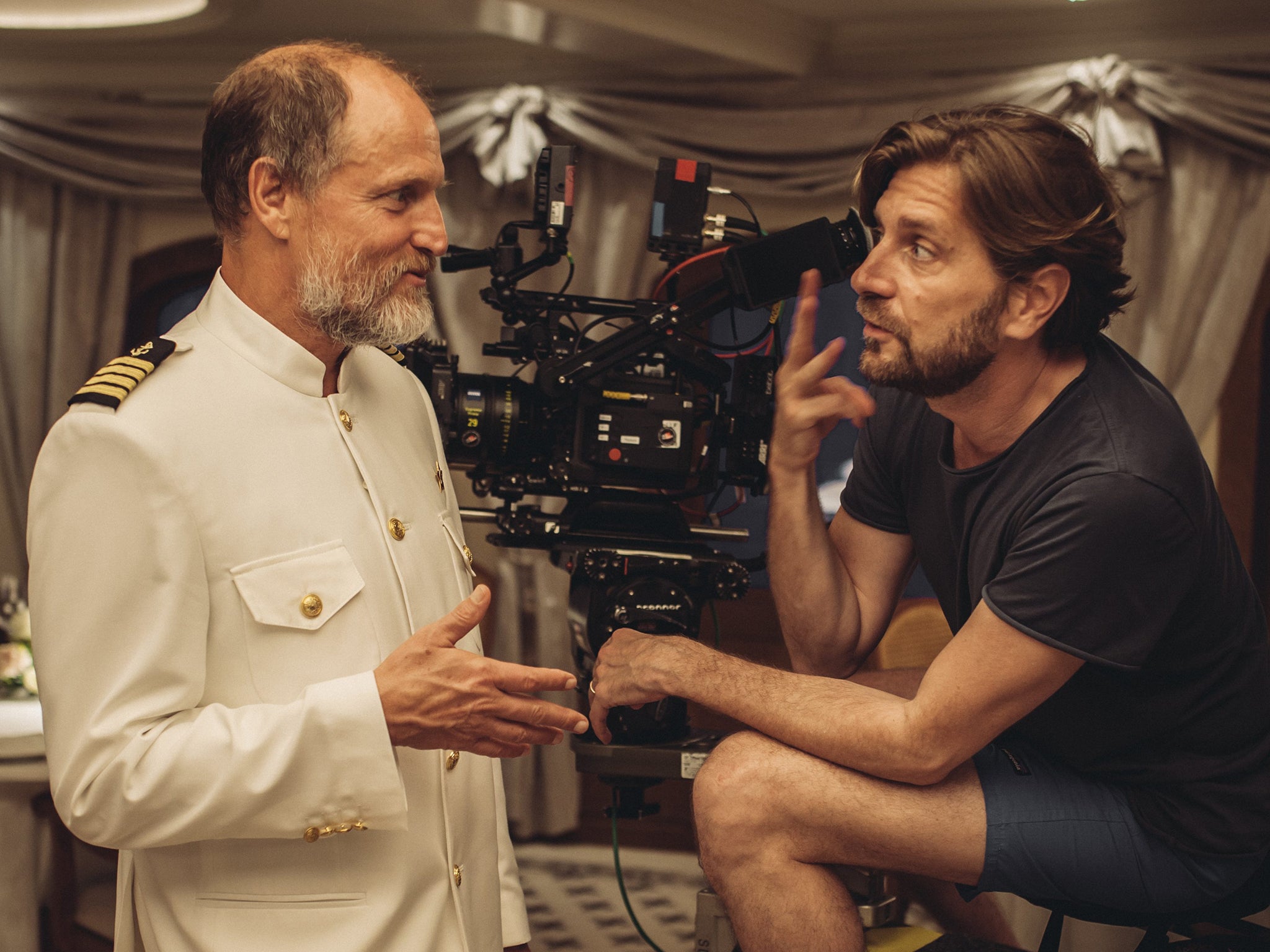In the detailed image, it captures actor Woody Harrelson in what seems to be a movie set. Woody Harrelson, positioned on the left, is distinguished by his balding middle and a scruffy white beard. He is dressed in a white jacket that resembles a ship captain or sailor uniform, complete with brass buttons and an anchor patch on the shoulder. Harrelson is engaged in conversation with a man on the right, who appears to be the director. The director, recognizable by his short brown hair, brown beard, black short-sleeved t-shirt, and blue shorts, is seated on a chair. Between them, a sophisticated black camera with various buttons and cords suggests a professional filming setup. In the background, light gray curtains adorn the windows, and the white floor shows gray patterns, adding to the organized setting. The setting suggests a detailed and controlled movie production environment with complex interactions and professional equipment.